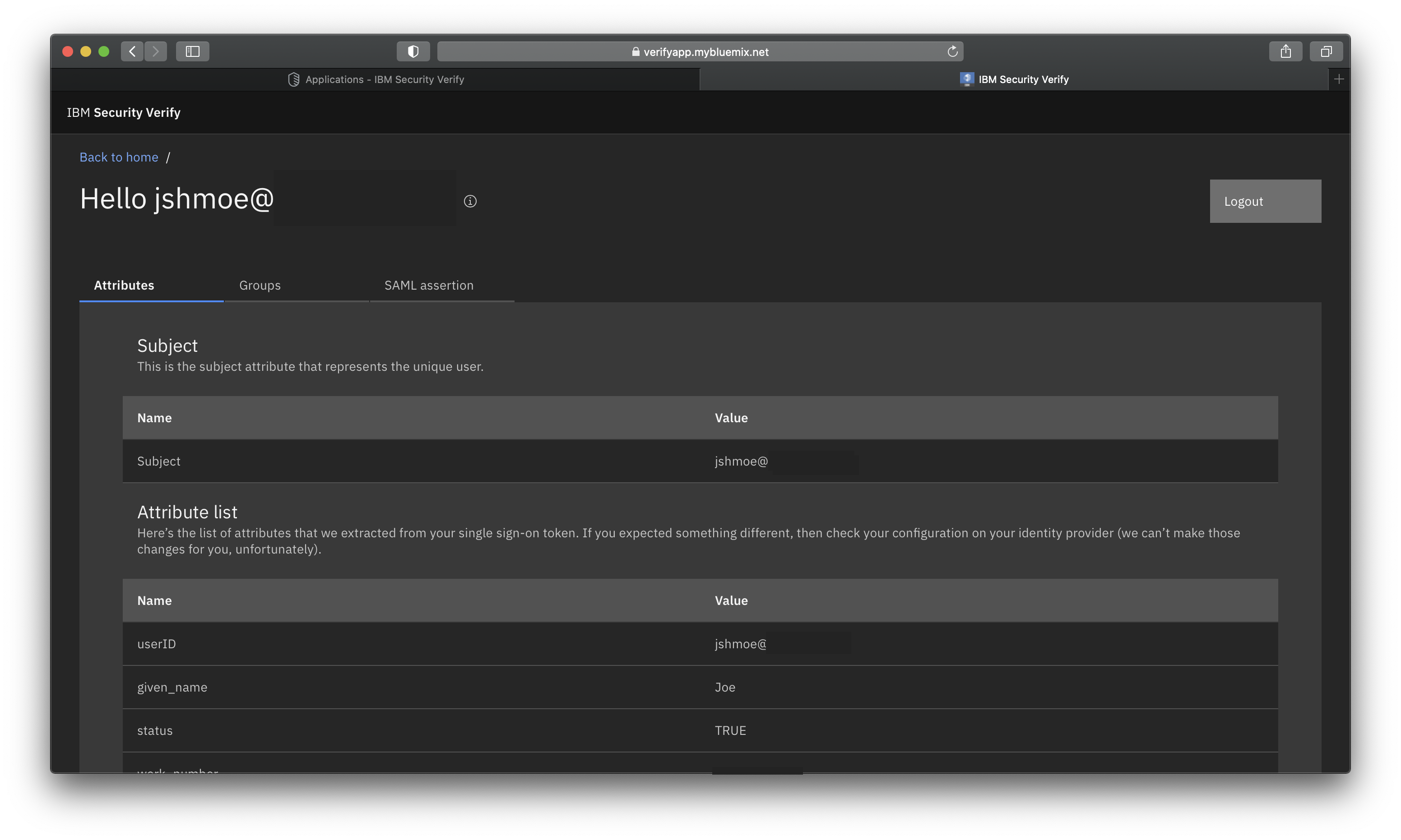This screenshot captures a segment of a website, which features a predominantly black and gray design. Although the URL at the top is somewhat obscured, it is discernible that it ends with ".net." At the very top of the page, the header prominently displays "IBM Security Verify" on both the left and right sides. Beneath this, a blue link labeled "Back to Home" is visible, and in white text, it greets the user as "Hello, J-S-H-M-O-E at," with a portion of the text redacted by a black rectangle. On the right-hand side of the header, there is a "Logout" button.

The main content area of the webpage is organized into three tabs: Attributes, Groups, and SAML Assertion. The Attributes tab is currently selected, which is indicated by a blue underline. The page details start with a section labeled "Subject," which notes that this attribute represents the unique user. Below this, in a list format, it outlines:

- **Name**: Subject
- **Value**: J-S-H-M-O-E at (with redacted information)

Further down, there is a section titled "Attributes List" that explains these are the attributes extracted from the user's single sign-on token. A notice advises users who anticipated different results to check their identity provider configuration since changes cannot be made from this interface. The text continues with additional details, but they are not fully captured in the provided description.